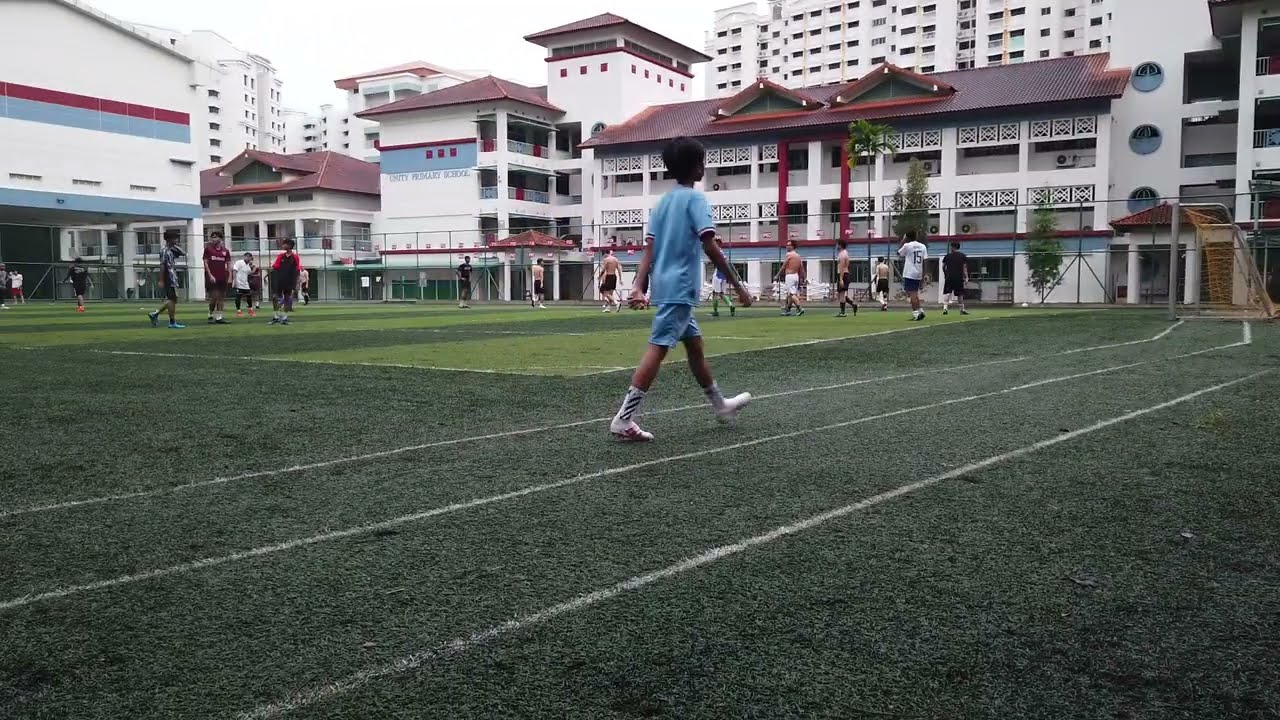The photograph, taken outdoors during the day, captures a vibrant scene at what appears to be a soccer field or track and field area, possibly in an Asian country. The foreground features a young boy, around 12 years old, with dark hair and dark skin, dressed in a blue jersey and shorts with white sneakers and socks, walking away from the viewer. The field is marked with white lines and includes a goal with an orange net on the right side. Scattered across the field are several people engaged in athletic activities, some in white shirts and others in black, suggesting a shirts versus skins game.

In the midground and background, the scene is framed by various structures. To the left, there is a tall, white building adorned with red and blue stripes. The central building boasts an Asian-inspired architectural style with a red roof and multiple gables, indicative of its location. Underneath a blue stripe on this building is the text "Unity Primary School." Further back, taller, multi-story white buildings, likely condos or office buildings, punctuate the skyline. The composition also includes a glimpse of the sky, with colors ranging from green and dark off-green to light blue, white, black, red, and brown, all contributing to the rich, detailed ambiance of this busy outdoor setting.